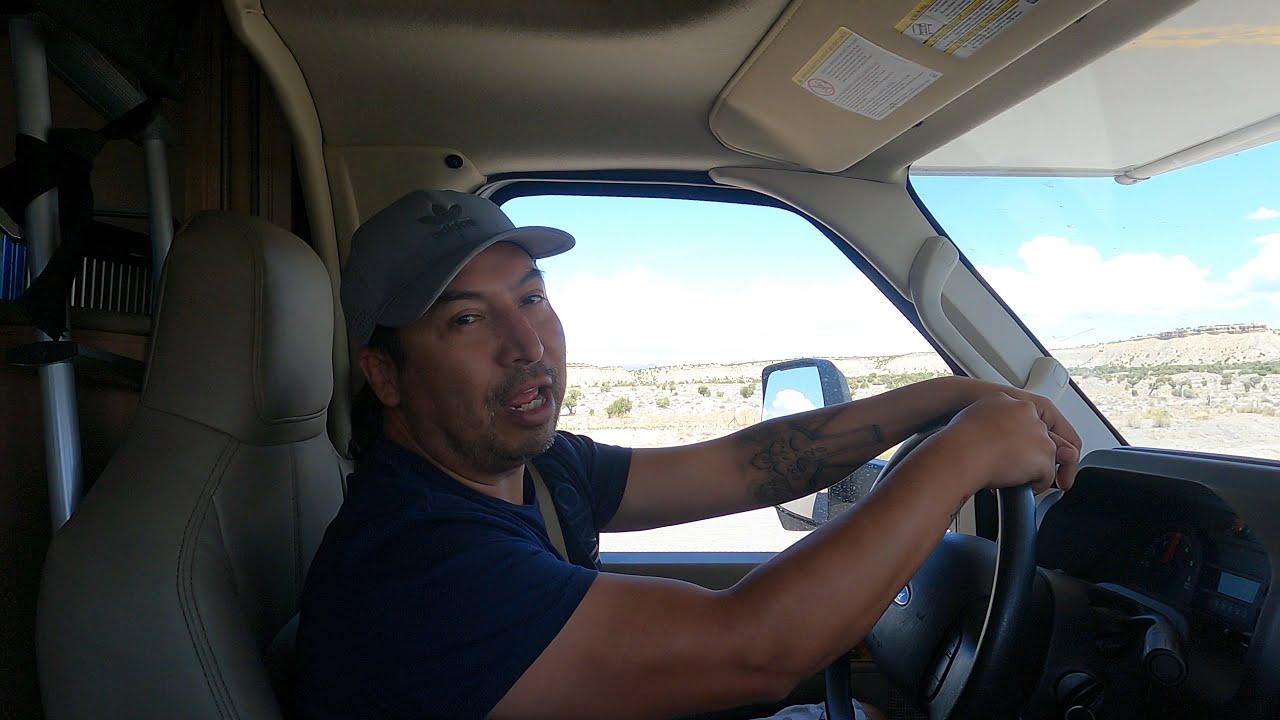The image depicts a close-up of a Hispanic man driving a large vehicle, possibly a truck or RV, through a desert landscape. The photo is taken from the passenger seat, capturing the driver, who is in his 30s or 40s, with dark skin and dark hair. He is looking towards the camera with his mouth partially open, as if talking. He is wearing a gray Adidas cap, a dark blue t-shirt, and has both hands on the steering wheel. Notably, he has a tattoo of an angel on his left forearm and is secured with a seatbelt. Inside the vehicle, the interior is all beige. Outside, the scenery features sand dunes with some vegetation under a bright blue sky adorned with fluffy white clouds.